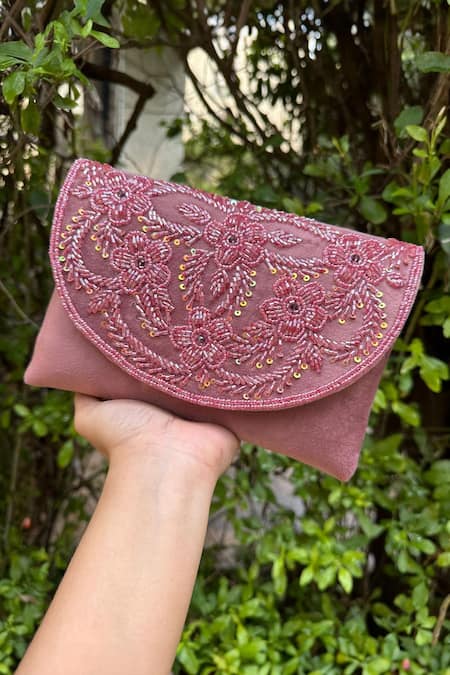In this photograph, the focal point is an elegant pink beaded purse held by a person with white skin. This handheld clutch is rendered in a velvety mauve with an intricate beaded and embroidered flap, showcasing detailed designs of paisley, flowers, and vines—all in various shades of pink. The person’s arm, visible from the wrist up, extends from the bottom left corner of the image, gripping the purse delicately. The backdrop of the scene is a lush green woodsy setting with an array of bright and dark green foliage. In the background, a white stone bridge can be seen, adding an additional layer of depth to the image. The purse exudes a feminine charm, making it a perfect accessory for pairing with a pink dress, a white dress, or any neutral-colored outfit.